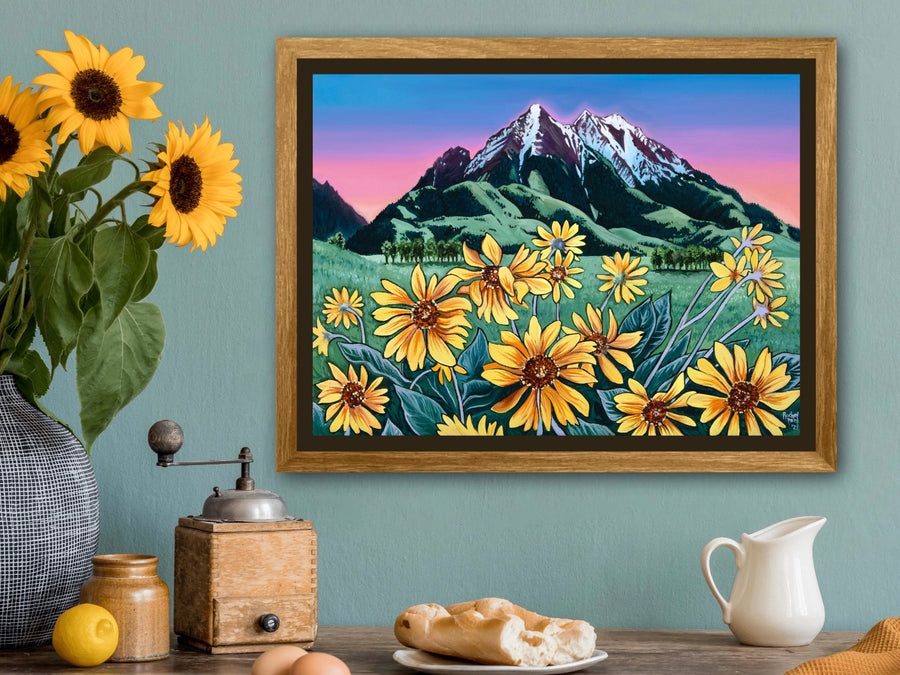The photo features a cozy corner of a home, set against a medium blue wall with hints of gray. Dominating the center background is a framed painting with a brown wooden frame. The painting captures a stunning landscape with a snow-capped mountain range under a dawn or dusk sky filled with hues of pink, purple, and blue. The foreground of the painting showcases vibrant sunflowers and rolling green hills with rows of distant trees.

In the left side of the image, there is a dark brown wooden table adorned with a few items. A gray vase holds three bright yellow sunflowers with dark green leaves, adding a touch of nature to the scene. Next to the vase sits a small brown jar with a lemon placed beside it. On this table, there is also an old-style coffee grinder as well as two brown eggs.

The right side of the table features a white plate with slices of French bread and a small, white pitcher. There is also a brown cloth partially visible on this side. Centered on the table, a nostalgic wooden music box stands out, waiting to be played.

This charming and detailed scene is beautifully composed, evoking a sense of comfort and rustic charm.